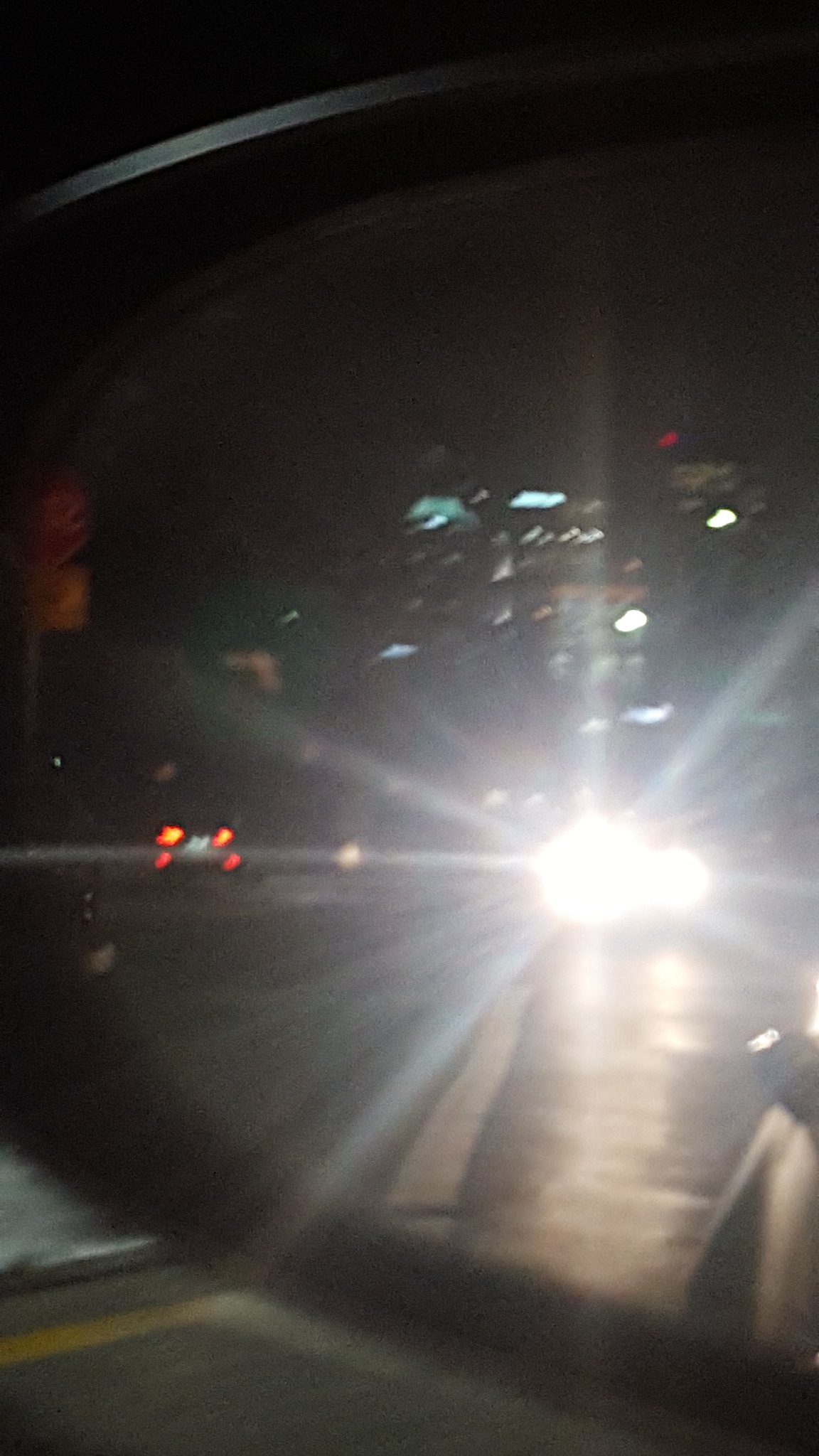The image appears to be taken from the perspective of a car's rearview mirror while in motion, making it somewhat challenging to discern specific details. The focal point is the glaring headlights of a car behind, emitting intense rays of light that dominate the center of the image, creating prominent lines. In the background, there are several buildings that resemble office spaces, suggesting an urban setting. Additionally, the brake lights of a car ahead are visible, hinting at a line of traffic. The overall scene is captured at night, as evidenced by the dark surroundings.